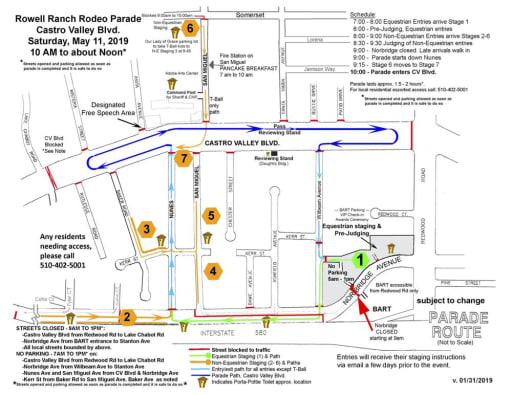This image is a square, multi-color print map with no border, and a white background. At the top left, in black text, it announces the Rowell Ranch Rodeo Parade on Castro Valley Blvd, scheduled for Saturday, May 11, 2019, from 10 a.m. to noon. The central feature of the map is Castro Valley Blvd, the main street of the town, depicted with various colored arrows outlining the parade route. Specific segments of the route are marked with blue, red, neon green, light blue, royal blue, and yellow arrows, indicating different groups and directions. The map includes several numbered locations, from 1 to 7, with number 1 prominently displayed in a neon green circle. While a key explaining these numbers exists, it is too small to read clearly. The lower right-hand corner of the map features the note: "Subject to Change, Parade Route."